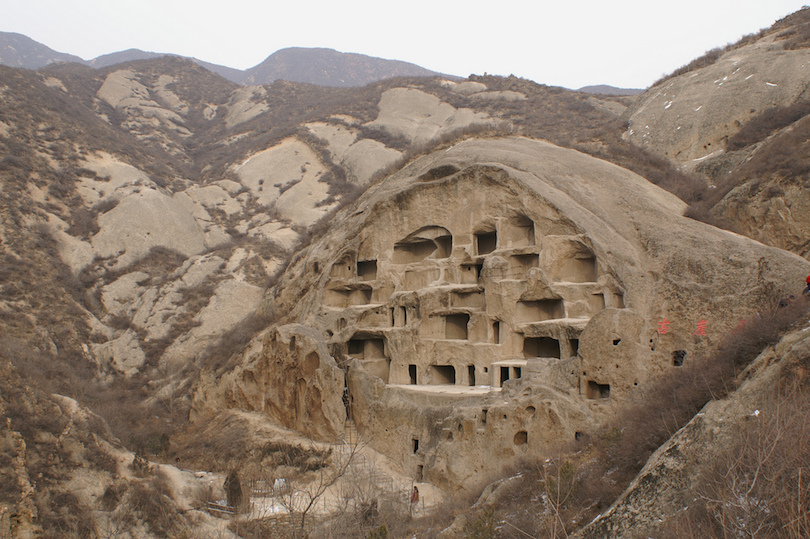This photograph captures an intricate and historical village carved directly into the side of a large, rocky mountain. The mountain itself descends towards the viewer from the top ridges at the upper left and right, with another mountain visible in the background under a clear sky. The ground at the base is covered in a pale, sandy dirt.

The carved structure comprises multiple dwellings, each featuring rectangular and square openings that resemble windows and doors, neatly arranged in five rows. These openings serve as entrances to different areas within the mountain, creating a labyrinthine network of homes, possibly designed for multiple families. 

Adding a sense of life to the image, a set of stairs carved into the rock leads down from one of these openings, and a person is seen walking down, emphasizing the human scale and functionality of this ancient dwelling. The facade of the structure is adorned with Japanese or Korean characters, hinting at the cultural and historical context of this remarkable mountainside village.